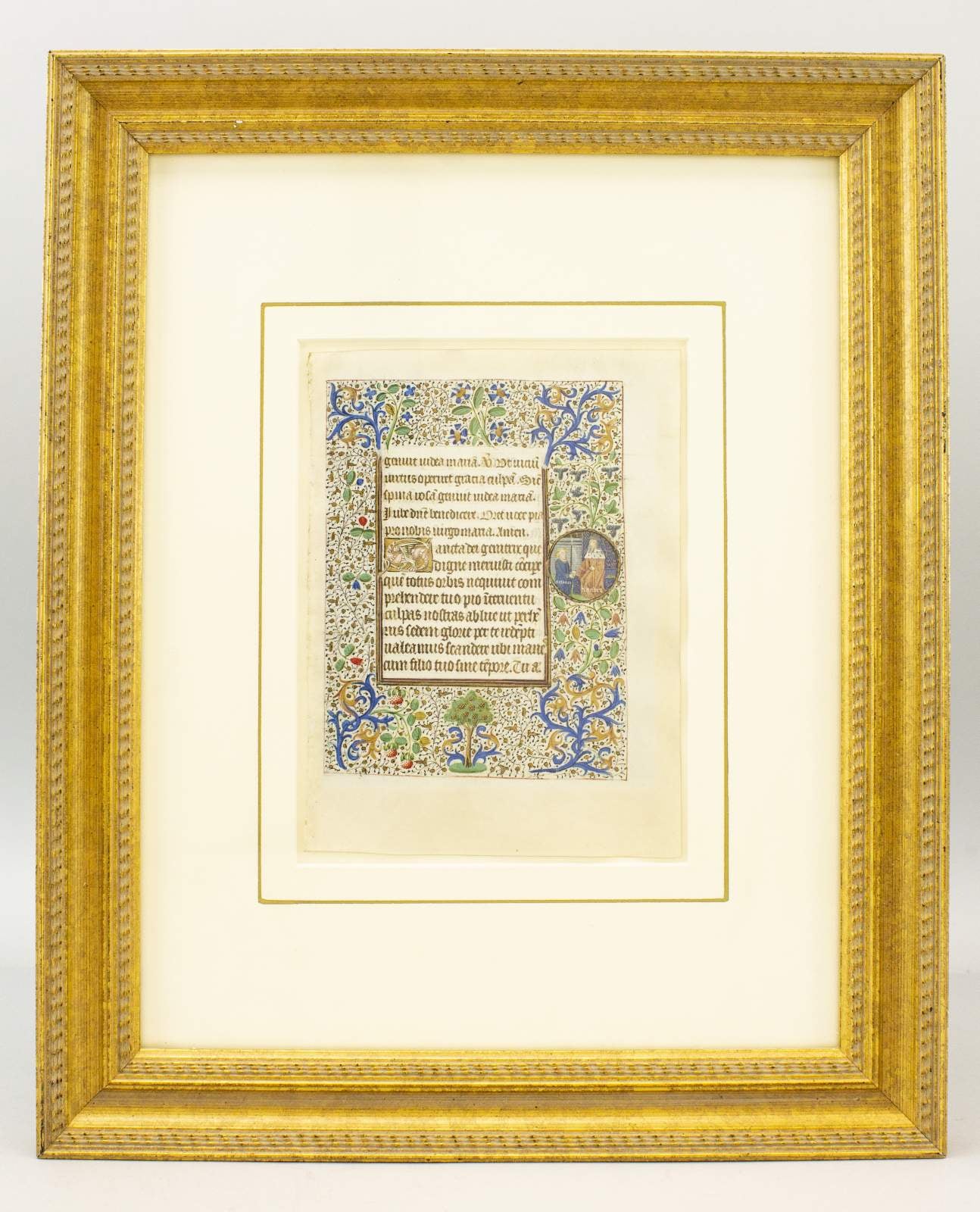The photograph shows a vertically-oriented, thick golden rectangular photo frame attached to a wall, enclosing a weathered, cream-colored page that appears to be from an old book. The frame's border is textured and about an inch and a half to two inches thick. Inside the frame, a wide cream-colored matting provides an elegant border, with an additional, thinner gold matting outlining the central item. The centerpiece of this framed display is a piece of paper featuring intricately stylized, handwritten or printed text in an indiscernible foreign language, likely Latin, surrounded by colorful decorations. The intricate designs include leaves, plants, and blue lines, rendered in green, orange, and blue hues. A prominent circular picture within the design depicts what appears to be two human figures. The entire piece is artistically matted against a slightly darker background, creating a stunning, vintage visual effect.